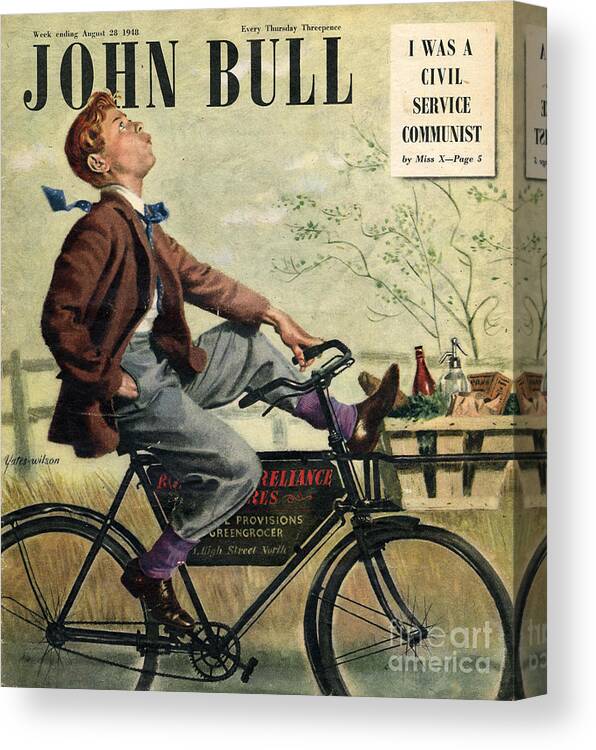The image, evocative of a Norman Rockwell painting, resembles the cover of a vintage John Bull magazine. Set against a nostalgic mid-20th century backdrop, it features a young man attired in a blue jacket, brown shoes, gray pants, purple socks, a white dress shirt, and a tie. He is leisurely riding a bicycle with a basket of food at the front, whistling and looking skyward. His right hand is casually tucked in his pocket, while his left hand grips the handlebars, and one foot rests on the bike's frame. The scene behind him includes a grassy area, a wooden post fence, and a picnic table adorned with food. The magazine's cover text, prominently displayed, reads "Week ending August 28, 1948, Every Thursday, 3 pence, John Bull." The upper right corner features a white rectangle with the inscription, "I was a civil service communist, by Ms. X, page 5."